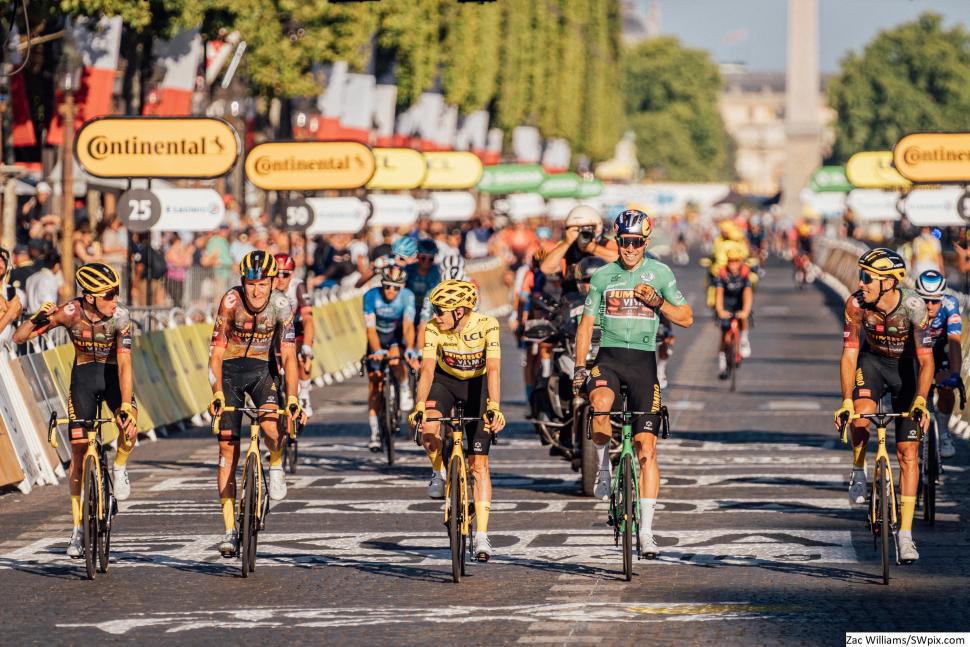In this vibrant landscape photo of a bike race, five cyclists dominate the foreground as they ride towards the camera, appearing to have just crossed the finish line. Each rider sports a distinctive, brightly colored outfit, and most wear yellow and black striped helmets. The man at the center, the most prominent rider, wears a green shirt, black pants, and a silver helmet, smiling broadly behind his glasses. To his left, a woman in a yellow shirt, matching yellow helmet, and bike looks to the side, while next to her, a man in an orange and gray shirt rides a yellow bike, also donning a yellow and black helmet. Another rider, further left, raises his fist in victory, sharing the same yellow and black helmet theme.

The blurred background accents the sharp focus on these joyful racers, teeming with green trees under the bright sunlight and featuring a white monument. Spectators lining the street behind barricades add to the race's lively atmosphere. The road is gray with white lettering, and yellow oval signs saying "Continental" are prominent along the track. In the bottom right corner, the photo is credited to Zach Williams at SWPIX.com.